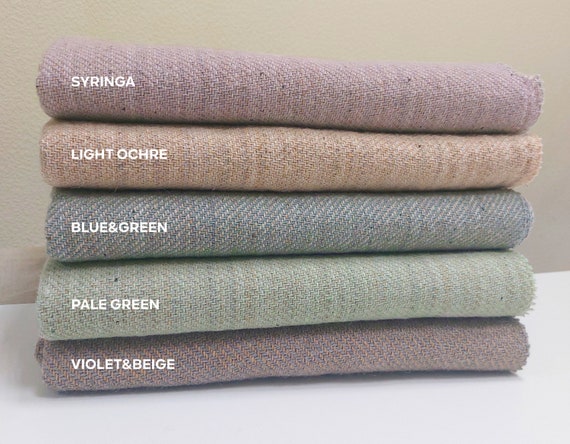This image is a detailed photograph of five neatly stacked fabrics or towels, wrapped around a core, displayed on a white surface against a cream-colored background. The fabrics, which appear to be part of an advertisement, are labeled with their respective colors in white capital letters. Starting from the top, the colors are syringa (a shade of purple), light ochre (a brown-bronzy hue), blue and green (a blend of blue and green), pale green (a soft green), and at the bottom, violet and beige (a mixture of violet and beige). Each fabric is made of thick material with heavy stitching, meticulously folded into a compact stack.